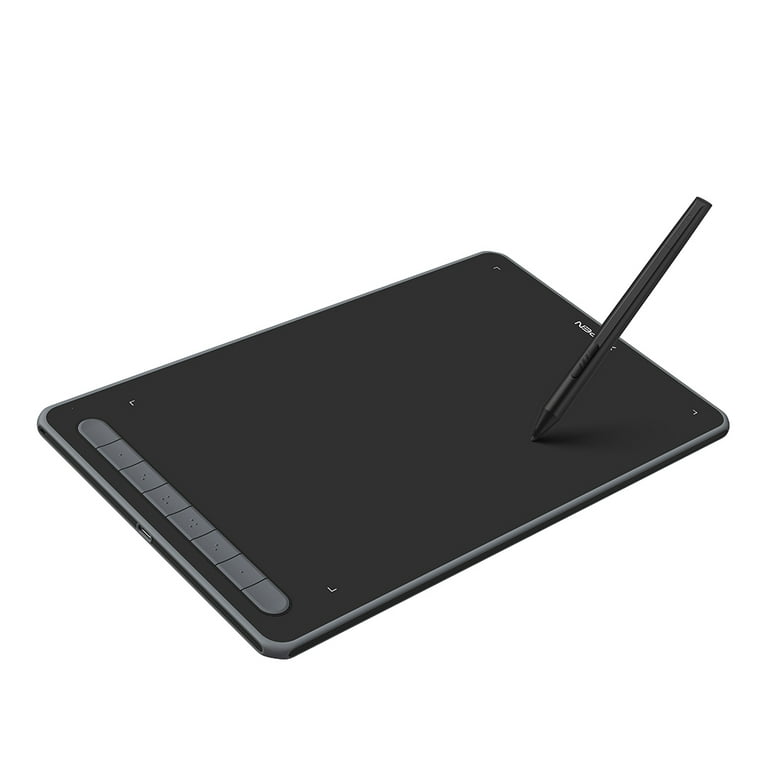This image showcases a black, rectangular electronic device, likely a tablet, set against a pristine white background. The device is angled diagonally, appearing upside down, with white text visible on what is now positioned as the upper right corner. A black pen, or stylus, rests against the tablet's surface, its tip lightly touching the device while standing at a diagonal angle. The tablet also features a row of eight gray buttons at one end, each marked with raised dots resembling Braille. The overall setup emphasizes the stark contrast between the black device and the solid white background, highlighting the sleek design and tactile features of the tablet.